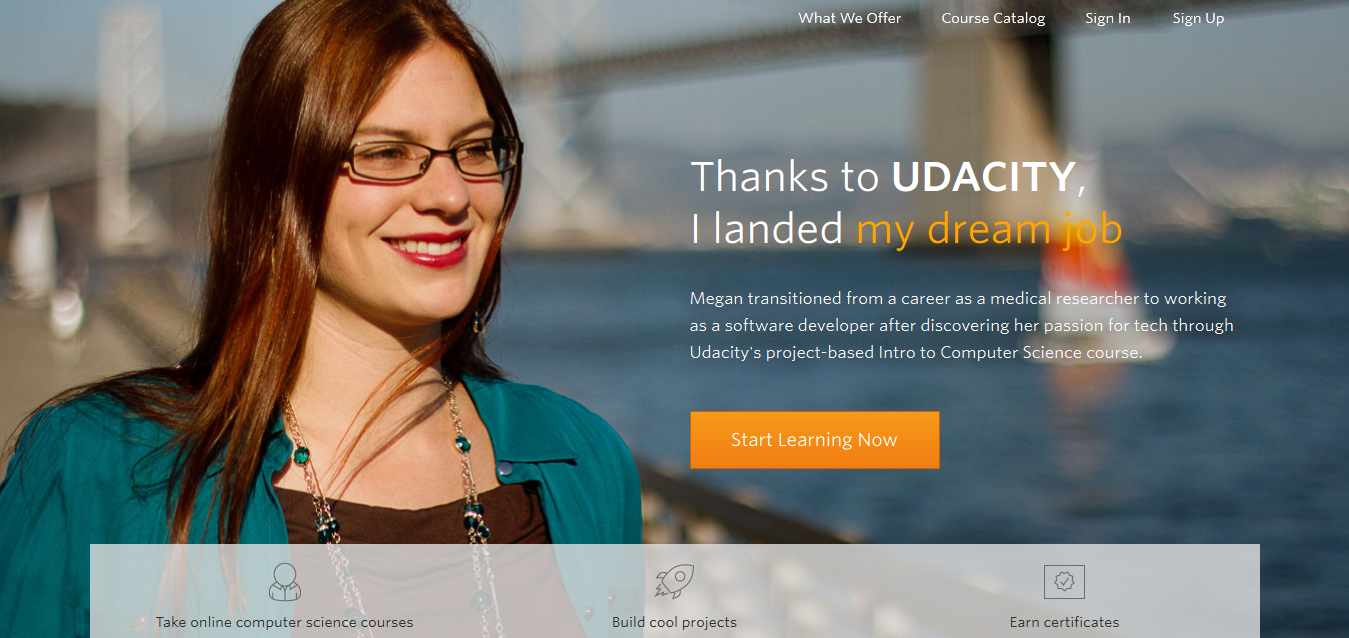The homepage of the website features a visually engaging background that spans the entire screen, centered around a high-resolution image. On the left side of the background image stands a woman with long brown hair, wearing glasses, red lipstick, and a turquoise top layered over a black undershirt. She accessorizes with a long gold necklace adorned with green rubies. The woman, smiling and gazing to her right, stands on what appears to be a boardwalk. Behind her, the out-of-focus background reveals a wide-angle view of a pier and bridge, extending horizontally across the composition with water visible to her right.

At the top right of the page, the navigation menu offers clickable categories: "What We Offer," "Course Catalog," "Sign In," and "Sign Up." Below this menu, a prominent headline is displayed in white text, reading, "Thanks to Udacity, I landed my dream job." The phrase "my dream job" stands out in orange. Underneath this headline is a brief paragraph in white text that shares a success story. Following the text is a prominent orange rectangular button labeled "Start Learning Now."

The bottom of the homepage features a semi-transparent grey footer overlay. This footer contains three icons with accompanying text descriptions. The left icon states "Take online computer science courses," the center icon promotes "Build cool projects," and the right icon encourages users to "Earn certificates."